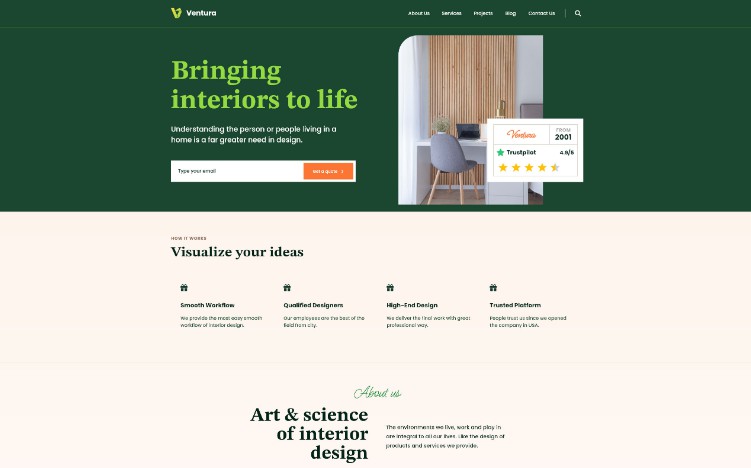The homepage of the Ventura website features a sleek and professional design. The upper half of the page has a dark green background. In the upper left corner, you’ll find the Ventura logo, a light green 'V', followed by the name 'Ventura' in white lettering. On the right side, there are several white links for navigation and a search icon represented by a magnifying glass.

Just below, a central image displays an office setup accompanied by the text "Ventura since 2001" and a Trustpilot rating of 4.8 out of 5 stars, visually represented by star icons filled to reflect this rating. To the left of the image, in light green text, it states "Bringing interiors to life," followed by a white text slogan: "Understanding the person or people living in a home is fundamental to great design."

Beneath this, a call-to-action invites users to enter their email address and click an orange button to book a consultation with Ventura interior designers.

The remainder of the website features a white background with black text, outlining various sections: "How it works," "Visualize your ideas," "Smooth workflow," "Qualified designers," "High-end design," and "Trusted platform." At the bottom of the page, there’s a section titled "About Us" along with a blurb detailing the company and its commitment to the art and science of interior design.